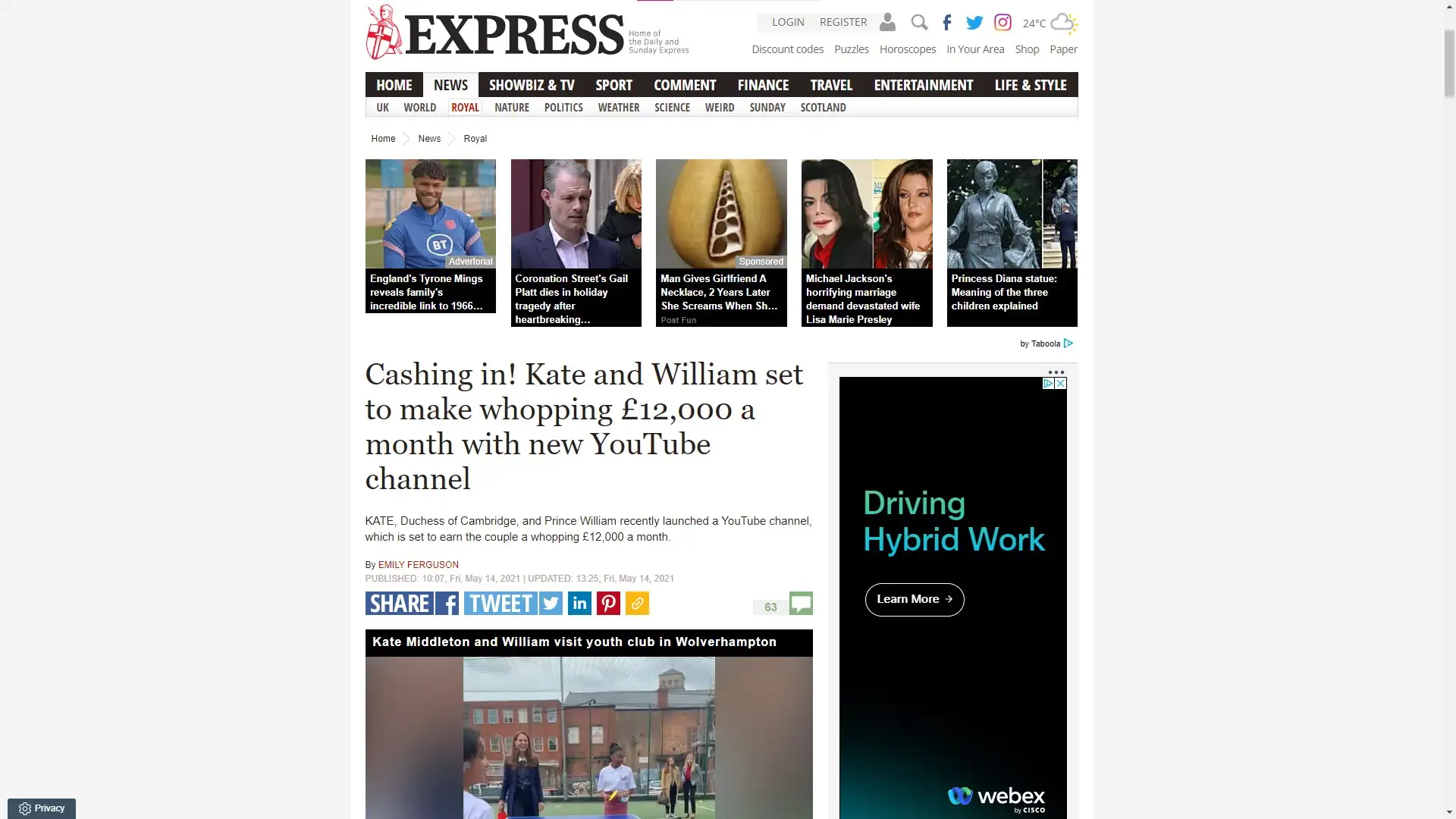The web page shown belongs to a news outlet named "Express." Situated in the upper left corner is the Express logo, which features a red and white medieval knight holding a shield. Adjacent to the logo, the word "Express" is prominently displayed in uppercase black font. In the upper right corner, the site provides links to additional resources, including a weather app, photos, Twitter, Facebook, and a search icon.

Underneath these top elements, there is a navigation bar offering various links for users to explore different sections of the website. This includes categories such as Home, News, Showbiz & TV, Sport, Comment, Finance, Travel, Entertainment, and Life & Style, with the "News" section currently active. The News section highlights five stories for readers to view.

Highlighted prominently beneath these categories is a news headline: "Cashing In: Kate and William Set to Make a Whopping £12,000 a Month with New YouTube Channel."